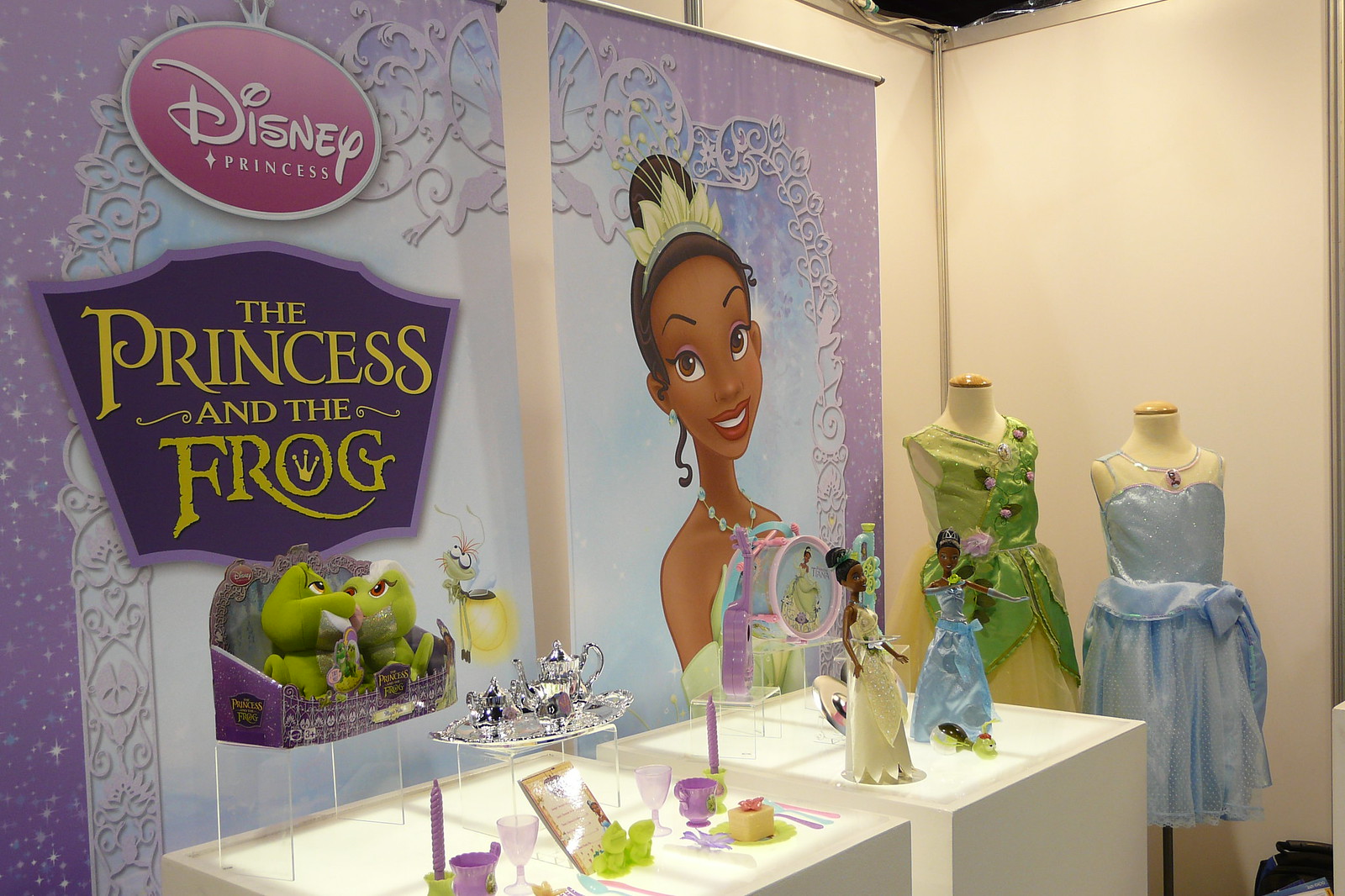The image depicts a detailed indoor display dedicated to Disney's "The Princess and the Frog," prominently featuring the first African-American Disney princess. The back wall showcases two banners: the left banner bears the Disney logo and the title "The Princess and the Frog," complemented by two plush frogs looking at each other. The right banner features an image of the African-American princess herself. In front of these banners, two headless mannequins display costumes: one in a green dress reminiscent of Tiana’s iconic gown and the other in a light blue dress. Additionally, there is a white display box adorned with a silver tea set, purple candles, and a box holding two green frog plush toys. A neighboring display box contains two dolls dressed in different gowns, reinforcing the regal theme. Furthermore, a tea set with desserts, which appear realistic but are actually faux, enhances the elaborate exhibit.